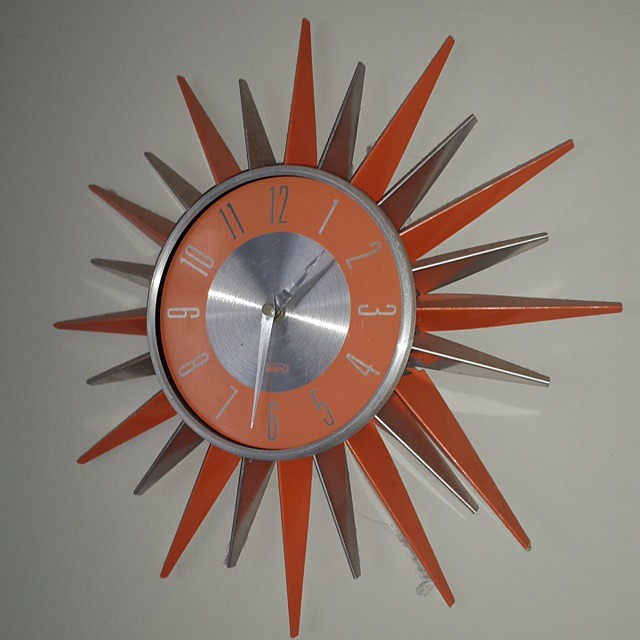This image showcases a clock hanging on a plain white wall, captured in a medium-quality photograph likely taken a few years ago with a phone or camera. The clock features a distinctive design with a silver outer border and an inner ring where the numbers are displayed in silver against an orange background. The center of the clock, where the hands are located, is also silver. The clock hands include a small and a long silver hand, both pointed. Surrounding the clock face are alternating long, pointy orange spikes and shorter bluish-black spikes, reminiscent of sun rays, that extend outward and form a pattern. The orange spikes align with the numbers on the clock, while the bluish-black spikes are positioned in between the numbers, creating a visually striking radial design.